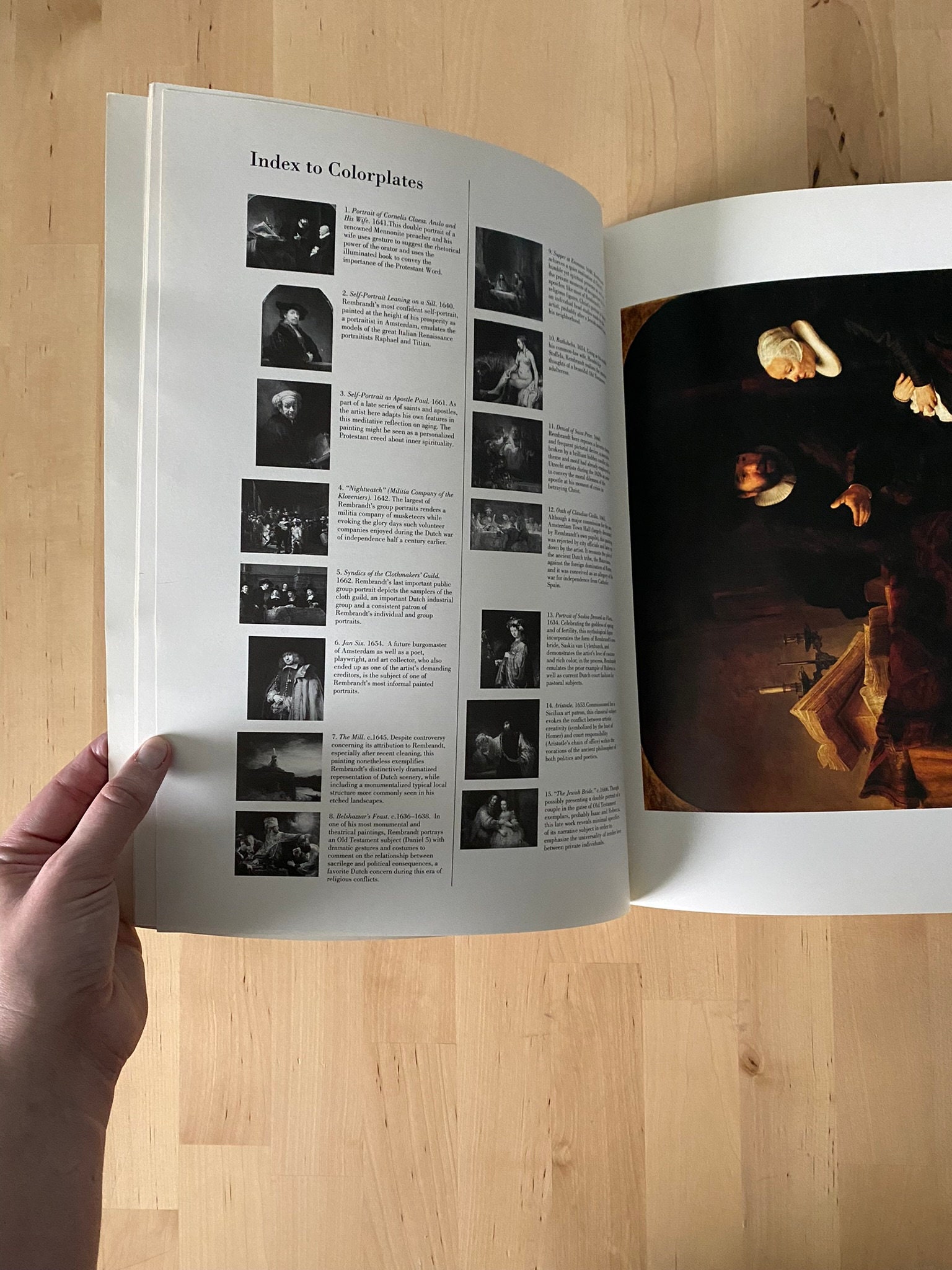In the photograph, we see a person's left hand holding open a large book with white pages. At the top of the left page, it reads "Index to Color Plates." This page features two columns, each with around eight black-and-white artistic images that appear to be from a classical era, possibly dating back to the 1700s or 1800s. Each image is accompanied by descriptions such as "Portrait of Cornelia," "Self-Portrait Leaning on Desk," "Apostle Paul," and "Night Watch." The detailed hand holding the book reveals a Caucasian skin tone and rests on a wooden table made of planks, showcasing visible wood grains.

On the right page, there is a full-color plate capturing an old scene featuring two people dressed in period attire. The man, who has a dark beard and hair and wears a black jacket with a white collar, is engaged in conversation with a woman with white hair and a similar white collar. They are positioned near a desk or table adorned with old-fashioned candle holders containing candles, enhancing the historical ambiance. The entire composition suggests a rich blend of history and artistry, making the book a valuable resource for those seeking historical images or artistic references.